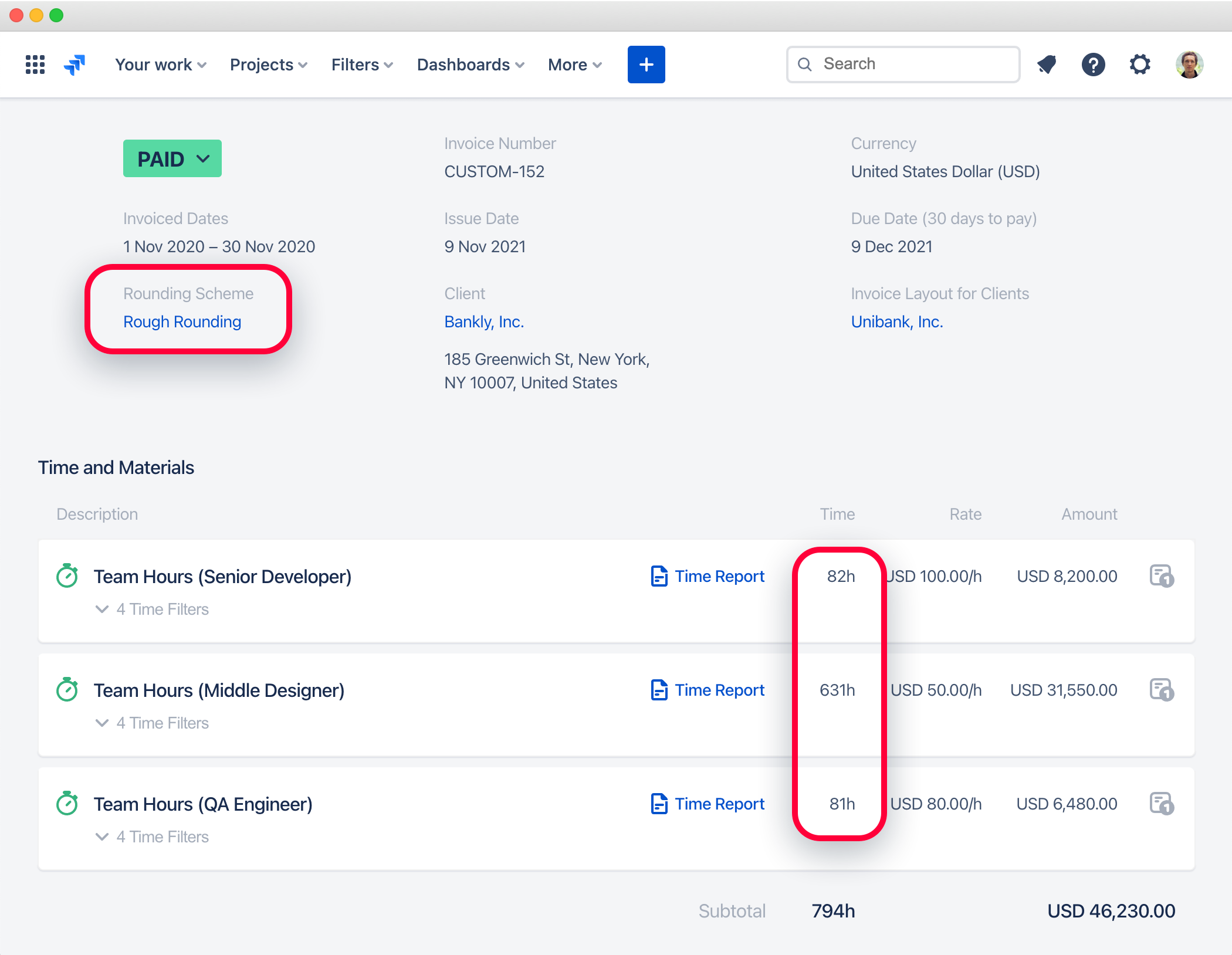This image appears to be a desktop screenshot of an Apple application focused on invoicing or project management. The user interface at the top features drop-down menus labeled 'Your Work', 'Projects', 'Filters', 'Dashboards', and 'More'. The main section of the page seems dedicated to a tutorial, as certain elements are highlighted with red circles or bubbles.

Central to the screen is a detailed invoice. The invoice status is marked as 'Paid', indicated by a green drop-down button that appears editable. The date range for the invoices is set between November 1st and November 30th, 2020. A highlighted note in red indicates a 'Rounding Scheme' named 'Rough Rounding'.

Additional invoice information includes:
- **Invoice Number**
- **Issue Date**
- **Currency**
- **Due Date**
- **Client's Location or Address**
- **Invoice Layout**

Items billed on the invoice are organized under 'Time and Materials', showcasing hours worked by different developers. A 'Time Report' link is available, which likely allows for downloading or viewing a detailed document. The hours worked by the developers are highlighted in red across one column, listing totals of 82 hours, 631 hours, and 81 hours, respectively. The corresponding rate and amount billed are also displayed, culminating in a subtotal for both the hours worked and the total amount due.

This well-structured view provides a comprehensive summary of the invoicing details, making it easier to track and manage financial transactions related to project work.